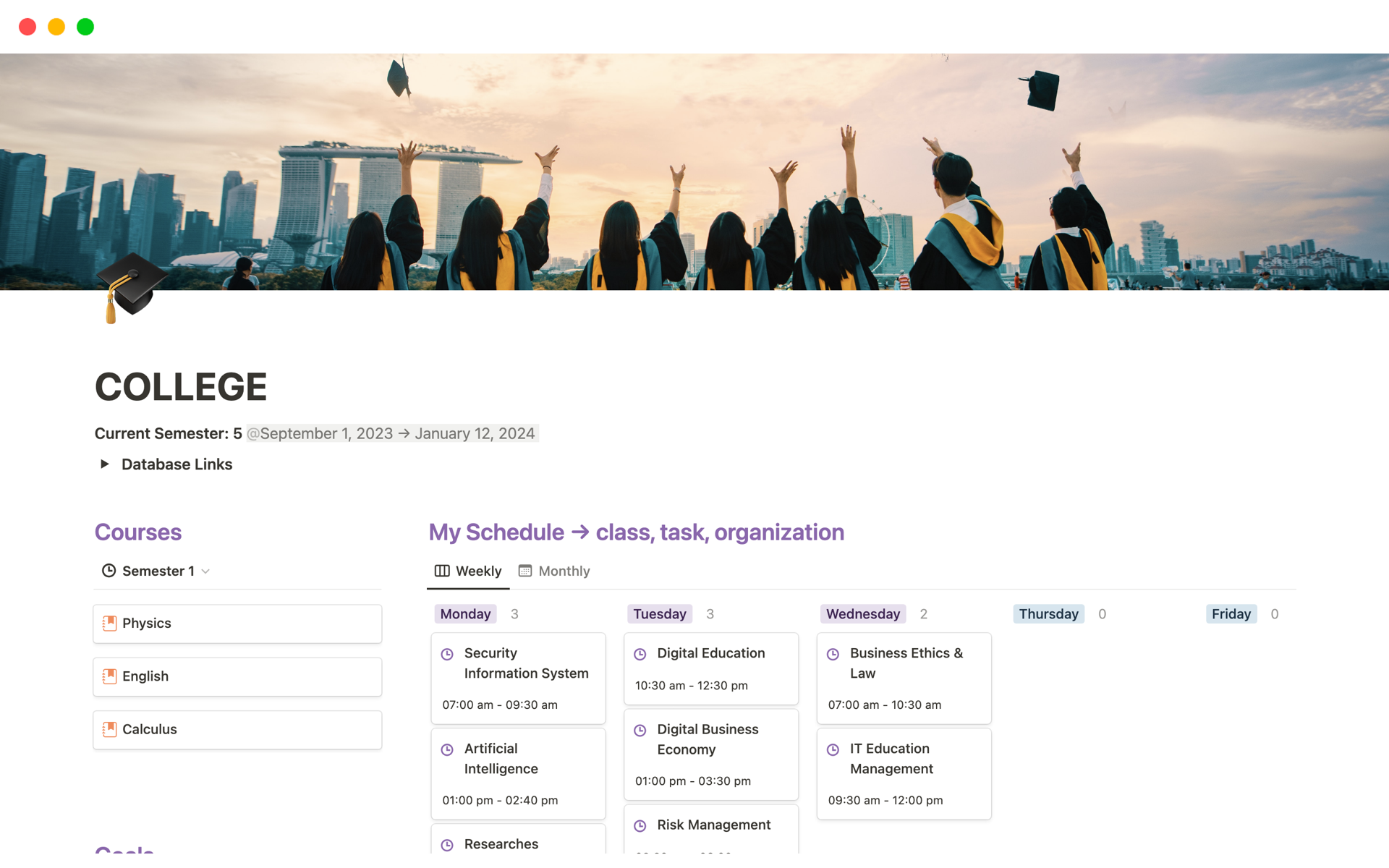The image depicts a college student's schedule organized for the current semester, starting from September 1st, 2023, and ending on January 12th, 2024. A prominent rectangular header at the top features an inspiring photo of graduates joyfully throwing their caps into the air against a backdrop of buildings and a clear sky.

Below the photo, the text confirms it as the "Current Semester 5" and includes functionality for "Database Links." The left side lists previous courses from Semester 1, which include Physics, English, and Calculus. The right side of the page is dedicated to the student's current schedule, organized under the categories "Class," "Task," and "Organization." The weekly schedule is highlighted in bold and underlined, but there is also an option to view it by the month.

The schedule breakdown is as follows:

- **Monday:** 
  - Security Information System: 7:00 AM - 9:30 AM
  - Artificial Intelligence: 1:00 PM - 2:40 PM
  - Research (time not fully visible)

- **Tuesday:** 
  - Digital Education: 10:30 AM - 12:30 PM
  - Digital Business Economy: 1:00 PM - 3:30 PM
  - Risk Management (time not fully visible)

- **Wednesday:** 
  - Business Ethics and Law: 7:00 AM - 10:30 AM
  - IT Education Management: 9:30 AM - 12:00 PM

The text across the top indicates the number of classes each day: `Monday - 3`, `Tuesday - 3`, `Wednesday - 2`, `Thursday - 0`, `Friday - 0`. This image appears to be from an app designed to help college students efficiently organize their classes and tasks, potentially offering reminders for when classes begin.